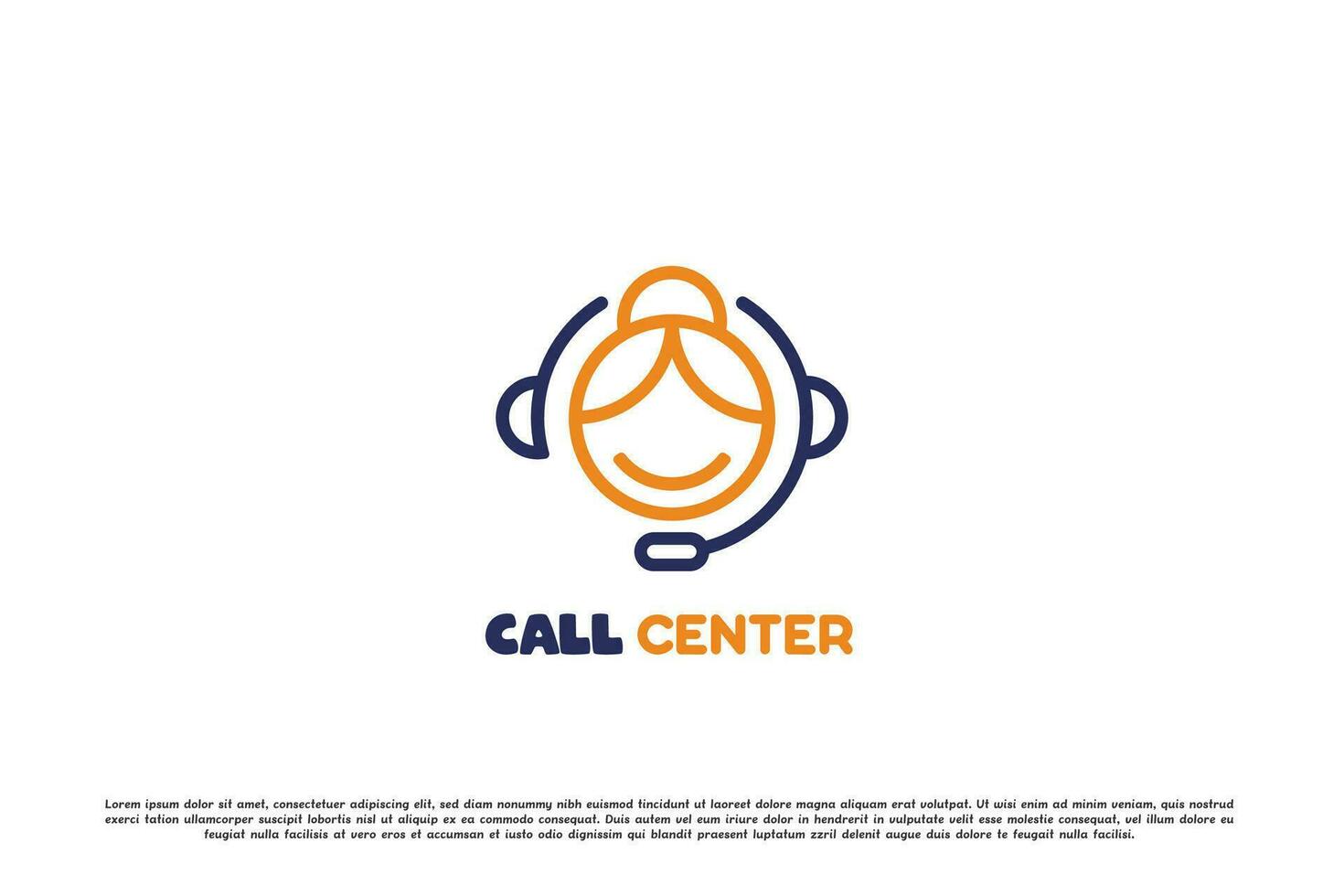The image is a logo for a call center, featuring a stylized, cartoon-like depiction of a woman's head and shoulders. Her face is minimalistic, with no eyes or nose, just a smile. Her hair is gold, parted down the middle, with bangs on both sides and a bun at the back. She is illustrated wearing a navy blue headset with a microphone extending from the left side. Below the image, the words "CALL CENTER" are written in all capital letters, with "CALL" in navy blue and "CENTER" in gold. There is also a paragraph of fine print beneath the main text, likely describing the call center, but the text is too small and possibly in a foreign language, making it unreadable.